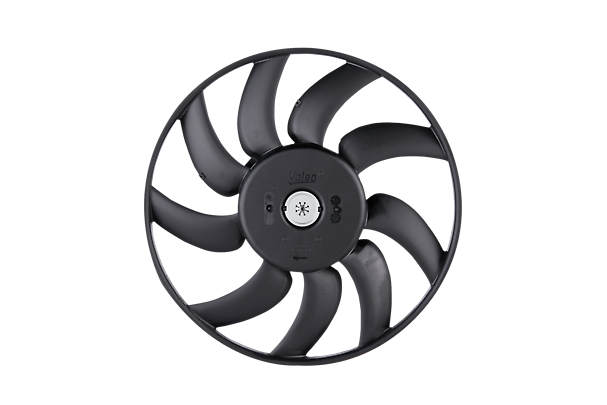The image depicts a detailed photograph of a black, heavy plastic fan component set against a pure white background, potentially useful in small machinery or computer systems. The circular fan features nine curved blades arranged diagonally, with a notable spacing discrepancy where the top five blades are closer together and the bottom four blades are similarly grouped, separated by slightly wider gaps. These blades connect an outer black plastic ring to an inner plastic donut-shaped piece. The central hub includes a metal cylinder and a silver disc, possibly for a battery, with the brand name "Valeo" stamped on it. Small text, indicative of settings or other information, as well as an arrow pointing left, are also visible on the thicker middle ring of the fan.